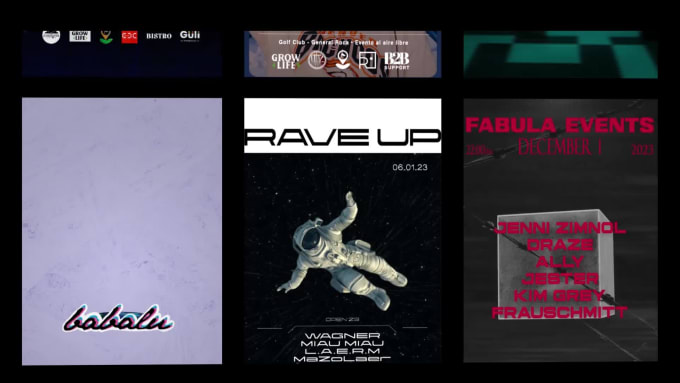The image is a black-themed poster, likely advertising a music festival or event. Central to the poster is a striking photograph of an astronaut in a white suit floating against the backdrop of space, with stars scattered around. Above the astronaut, bold black text reads "Rave Up 060123." Below the image, additional text features the names "Wagner," "Meow Meow," and "Muzzle Lar."

To the left of the central image, there's a rectangular section with a light purple background and black cursive text at the bottom saying "Babaloo." On the right side of the astronaut, another section appears with a dark gray background containing red text that reads "Fabula Events December 1, 2023." Below this are the names "Jenny Zimno," "Drez," "Allie," "Jester," "Kim Gray," and "Fro Schmitt." The overall design suggests multiple event promotions or contributors to the festival, with a visually engaging and modern aesthetic.